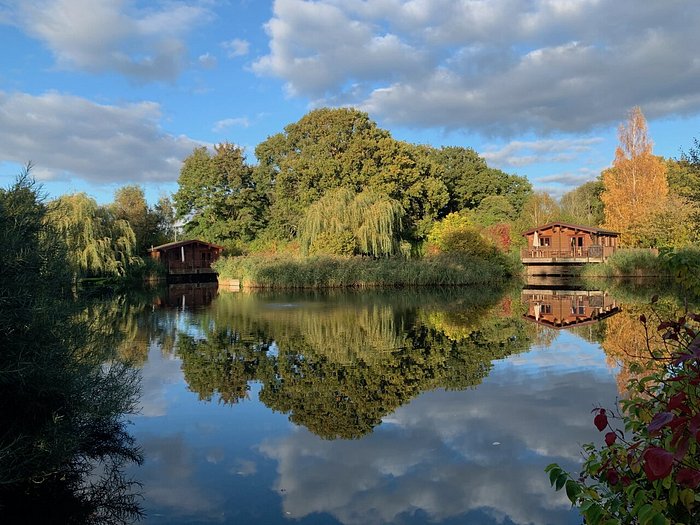This photograph captures a serene, picturesque scene in nature featuring a clear, tranquil lake reflecting its surroundings like a mirror. The lake, bordered by verdant, low-hanging willow trees and traditional bushy trees in greens and yellows with a smattering of autumnal oranges and reds, stretches out under a cloudy, light blue sky. On either side of the lake, nestled among the dense, reed-filled woods, stand two quaint wooden cabins with reddish-brown walls and brown roofs, each sporting a patio with an umbrella. The bright sunlight illuminates the trees, making them appear even more vibrant, while the bushes on the left remain in shadow. Delicate pink flowers peep out near green leaves in the foreground, adding a touch of color to the rich greenery. The absolute stillness of the lake creates a perfect, mirrored reflection of the trees, clouds, and cabins, emphasizing the pristine and undisturbed beauty of this natural landscape.